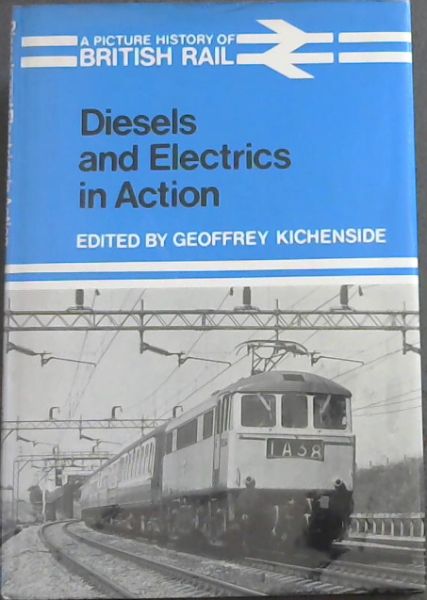The image depicts the cover of a book titled "A Picture History of British Rail," emphasizing a specific edition named "Diesels and Electrics in Action," edited by Geoffrey Kitchenside. The overall design features a light blue background for the upper half and a gray lower half. At the very top, in white text, it reads "A Picture History of British Rail," followed by the subtitle "Diesels and Electrics in Action" in black text, centered within the blue portion. Beneath this, also in white text, it says "Edited by Geoffrey Kitchenside." The lower half of the cover displays a black-and-white photograph of an electric train on the tracks. The train, numbered 1A38, is moving towards the viewer, and the image showcases wires and scaffolding overhead, indicating the electrical grid for the train. The photo has a retro feel, suggesting it is from the earlier part of the 20th century, and adds to the historical theme of the book.